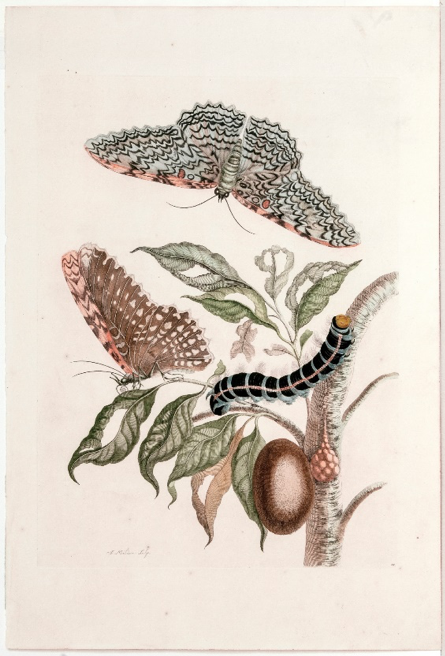The artwork depicts the intricate life cycle of a butterfly or moth, set against a pale, brownish-pink background bordered by a subtle gray edge. The vertically rectangular image includes various stages of metamorphosis, illustrated with detailed botanical elements like leaves, stems, and branches. At the lower right corner, a brown sack (a cocoon) hangs from a twig, with a black caterpillar featuring white lines visible on the branch. Additionally, there is an oval-shaped, nut-like structure nearby. On a green leaf, one butterfly rests with its wings folded, revealing brown, white, and possibly orange patterns that resemble those of a monarch. Meanwhile, at the very top, another butterfly, primarily white with black and orange markings, flies with its wings open as if descending. The beautifully textured wings display a repetitive up-and-down triangular pattern, showcasing the intricate artistry and attention to detail in illustrating this educational depiction of a butterfly's or moth's lifecycle.